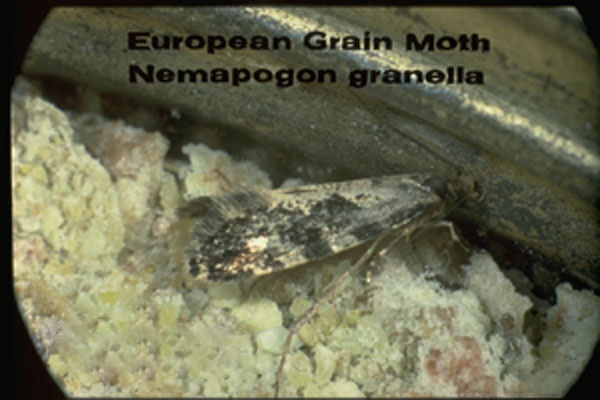This is a close-up, slightly blurry photograph of a European Grain Moth (Nemapogon granella), centered in the image. The moth is facing to the right, with its elongated body covered by closed wings that display a mottled pattern of black, gray, and white. It has two antennae and multiple legs resting on a rocky, yellowish pebbled ground. In the foreground, there appears to be a rusted, weathered metal beam, and to the side, a smooth wooden surface is visible. The image has a distinctive round shape with black curved edges and a black border. At the top of the photograph, in black text, it reads "European Grain Moth, Nemapogon granella."